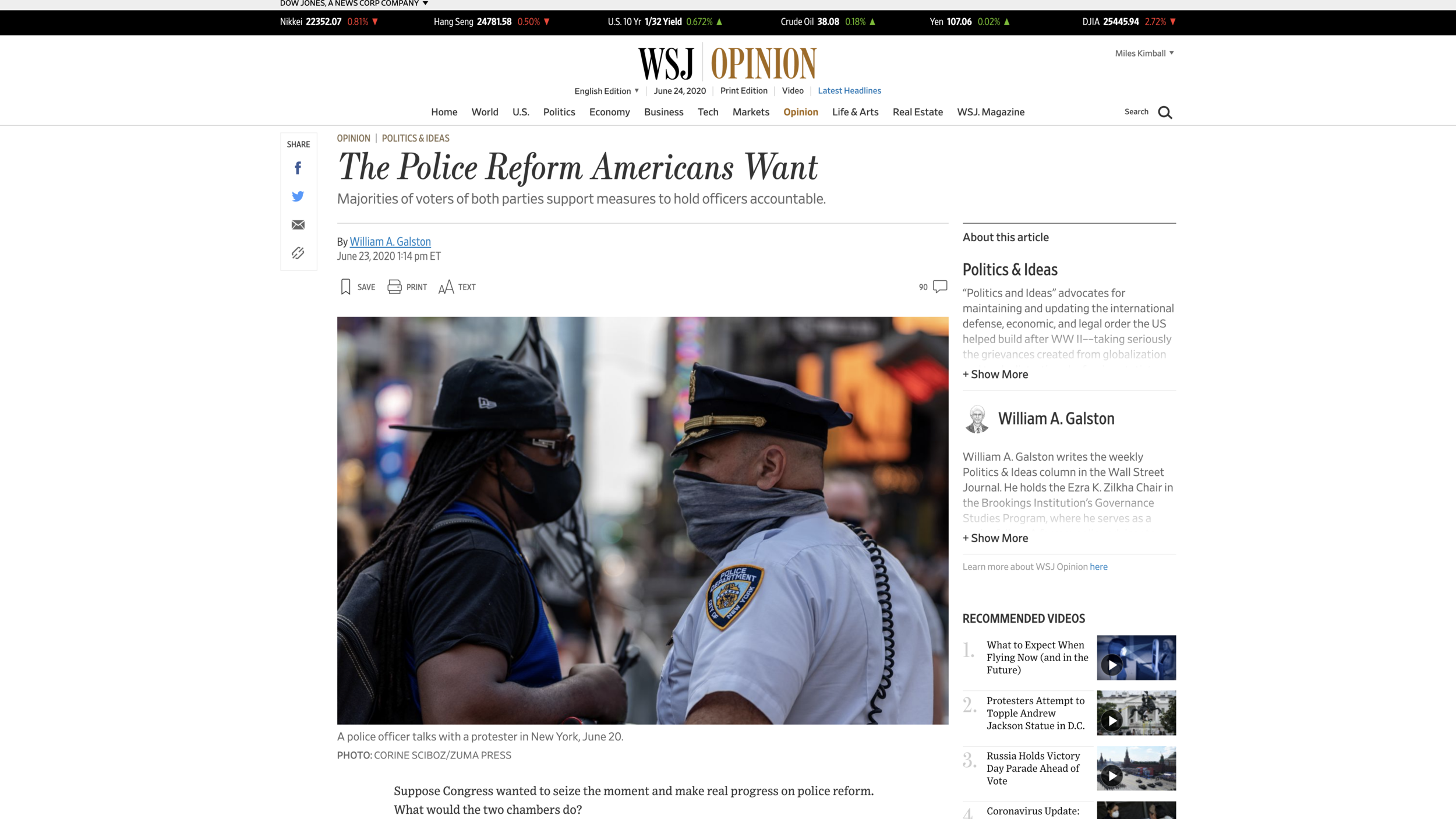A screen capture from the Wall Street Journal website prominently displays the black "WSJ" logo to the left, with the word "OPINION" in gold uppercase letters to the right. The main content of the image features an article with the headline "The Police Reform Americans Want," followed by the subheadline, "Majority of voters of both parties support measures to hold officers accountable."

The accompanying image depicts a tense face-off between a protester and a police officer. The protester, a Black man, is dressed entirely in black, including a mask, shades, a backward baseball cap, and a shirt. He also wears a blue safety vest. The police officer facing him wears a gray gator mask and a white shirt, with a visible radio cord running from his shoulder-mounted mic. Their intense stares suggest a potential confrontation. Below the image, the caption reads, "A police officer talks with a protester in New York, June 20th." At the very bottom of the screen, a question prompts readers: "Suppose Congress wanted to seize the moment and make real progress on police reform. What would the two chambers do?"